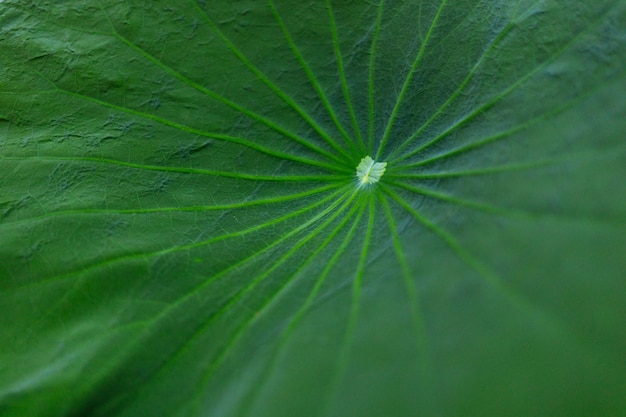This rectangular horizontal color image is an extreme close-up of a leaf, highlighted by a striking white feathery growth centrally located, just right and slightly above the middle. The leaf itself is a rich dark green, with additional detailed vein patterns scattered throughout. Emanating from the white center are about 20 medium green veins that spread outward in a starburst fashion, with the central veins lighter than the leaf and highlighted prominently. The photograph accentuates the leaf's texture, appearing almost papery, especially noticeable in the top-right and top-left areas. The bottom of the image blurs, making it more challenging to discern the intricate vein patterns and texture. The white central growth features a yellow core and expands into petal-like structures, suggesting the beginning of a blossoming flower, adding a touch of complexity and focal interest to the image.